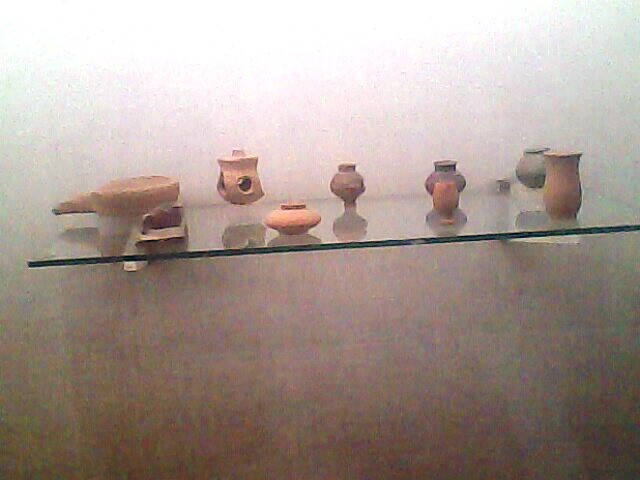The photograph captures a square image of a glass shelf mounted on the wall with metal brackets. Arranged neatly on the thick glass shelf are nine pieces of pottery, resembling small ancient artifacts. These ceramic works include pots, vases, and a possible cooking pan or pestle, all showcasing significant weathering that evokes the appearance of ancient stone artifacts with weathered edges. The pottery pieces vary in color from light brown and copper brown to dark brown. They are small, each measuring approximately two to three inches in height. The display features a combination of shapes: a short, fat one, several round ones—with some having necks, a bowl with a handle, and a jar-like piece with a lid featuring holes around the middle. The pieces are arranged in two rows, with five in the back and four in the front, all set against a light-colored wall that provides a clear and minimalistic background.